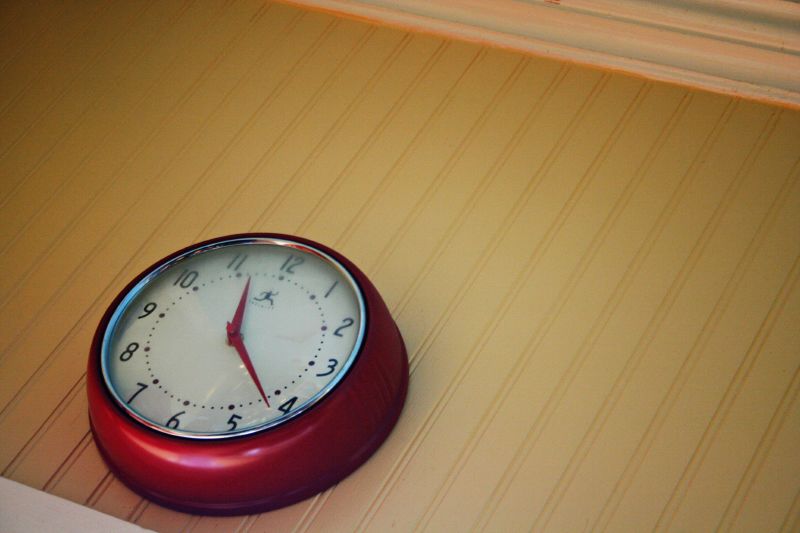This photograph captures a round clock mounted on a vibrant yellow wall, featuring textured indentation stripes for added visual depth. The clock, viewed from a low and steep upward angle, prominently extends from the wall with a bold red frame. Its white face displays standard numerals for timekeeping. Notably, just beneath the numeral 12, there is a small stick figure icon of a running man. The time indicated on the clock is approximately 11:21.